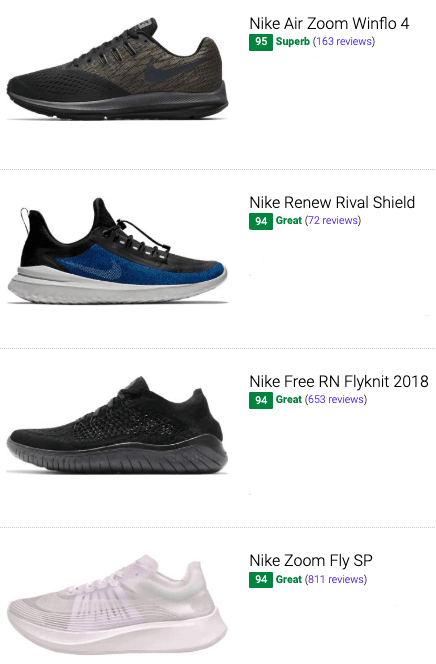The image appears to be a screenshot showcasing a selection of Nike shoes with accompanying details. There are four shoe listings, each displaying the side profile of the shoe:

1. The top shoe is facing left and is a dark brown color. It has a Nike checkmark that is partially visible and features a black mesh on the front. This model is labeled as "Nike Air Zoom Windflow". It is priced at $94.95, with the price highlighted in a green box and the "95" in white font. The shoe has a rating of "Superb" based on 163 reviews, which are displayed in purple font.

2. The second shoe is a combination of blue and black with a white sole, facing right. It is identified as the "Nike Renew Rival Shield". This shoe is priced at $94, also shown in a green box, and is rated as "Great" with 72 reviews.

3. The third shoe is an entirely black model, including the sole and shoelaces, facing left. It is named "Nike Free RN Flyknit 2018". This shoe is also priced at $94, contained within a green box, and carries a "Great" rating with 633 reviews.

4. The final shoe is a very light pink color, also facing left. It is labeled "Nike Zoom Fly SP". Like the others, it is priced at $94 and has a "Great" rating based on 811 reviews.

Each listing provides the model name, price, rating, and number of reviews, with all shoes displayed in side profile.